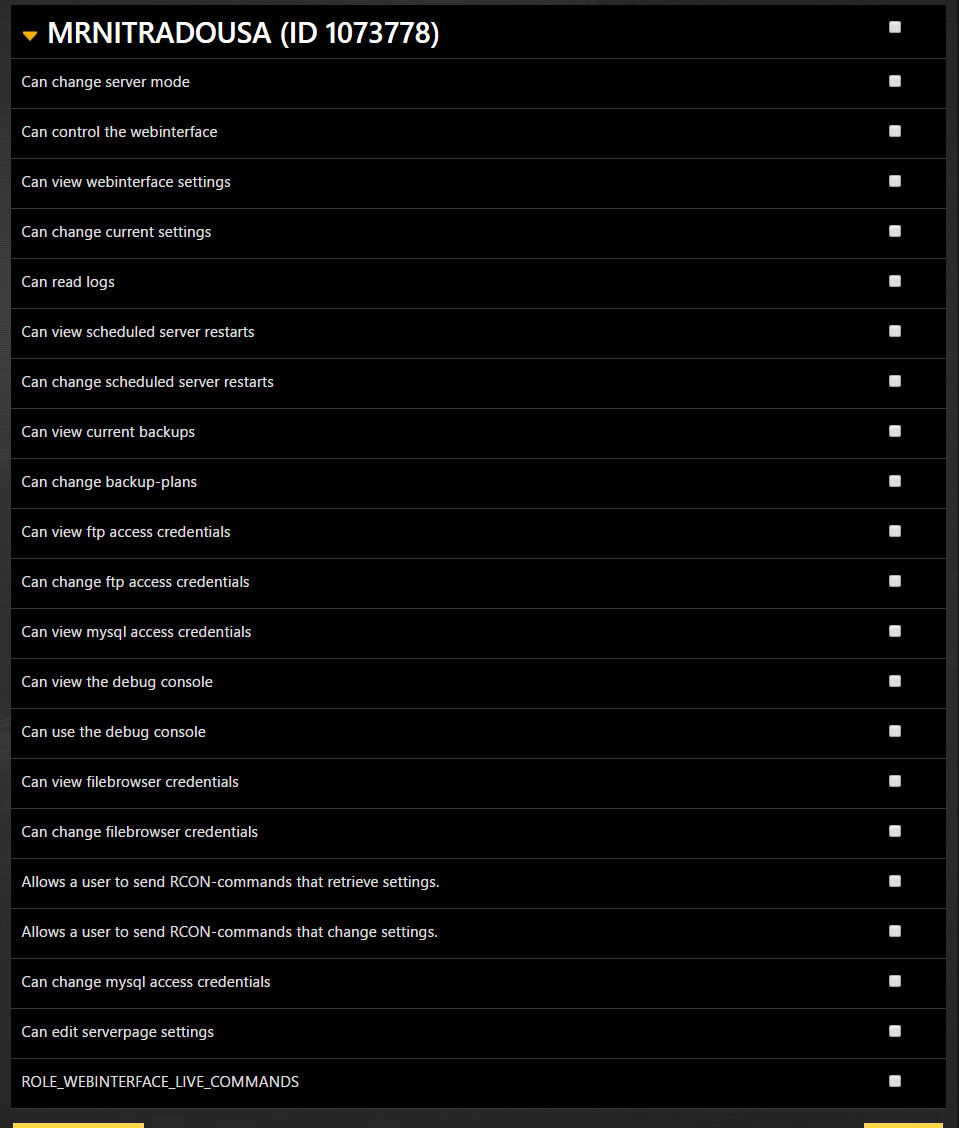The image depicts a large black rectangle divided into twenty-one sections by very faint gray lines. Each section represents a different setting. At the top of the rectangle, an orange downward-pointing triangle is labeled as "Mr. Nitra Dousa (ID: 1073778)" in uppercase letters. 

Each setting is accompanied by an unmarked white square, indicating that no settings have been selected. The list of settings includes:

1. Can change server mode
2. Can control the web interface
3. Can view web interface settings
4. Can change current settings
5. Can read logs
6. Can view scheduled server restarts
7. Can change scheduled server restarts
8. Can view current backups
9. Can change backup plans
10. Can view FTP access credentials
11. Can change FTP access credentials
12. Can view MySQL access credentials
13. Can view the debug console
14. Can use the debug console
15. Can view file browser credentials
16. Can change file browser credentials
17. Allows a user to send RCON commands that retrieve settings
18. Allows the user to send RCON commands that change settings
19. Can change MySQL access credentials
20. Can edit server page settings
21. ROLL_WEB_INTERFACE_LIVE_COMMANDS (written entirely in uppercase)

Finally, at the bottom of the page, two yellow bars are partially visible, indicating they may be cut off from the rest of the image. The white squares next to each setting are all empty, with no check marks or indicators selected.